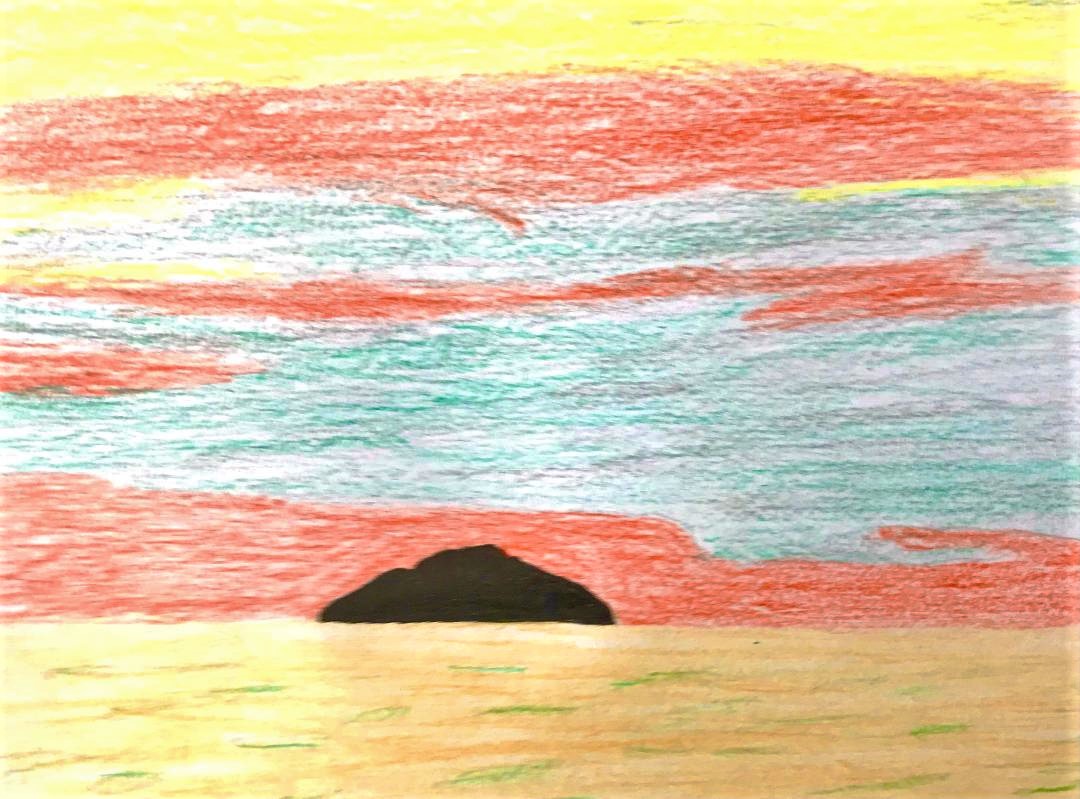This color photograph features a simplistic, childlike line drawing, likely created with crayons and markers. Central to the composition is an oval-shaped, deeply colored black object resembling an island. This "island" sits towards the lower center of the image. Below the island, a sea rendered in yellow and green waves is visible, suggesting a serene oceanic scene. Above the island, a red pencil-shaded area stretches across the drawing, transitioning to a gradient sky.

The sky is depicted with various color bands: an area of blue and grey follows the red pencilling, succeeded by another red line. A mixed-color line follows, with yellow to the left and blue towards the right, capped by a thicker red crayon stroke. At the very top of the image, yellow crayon coloring completes the sky. The island's intense black hue, possibly achieved with a marker, contrasts with the softer crayon textures of the sea and sky, creating a striking yet simplistic visual narrative.